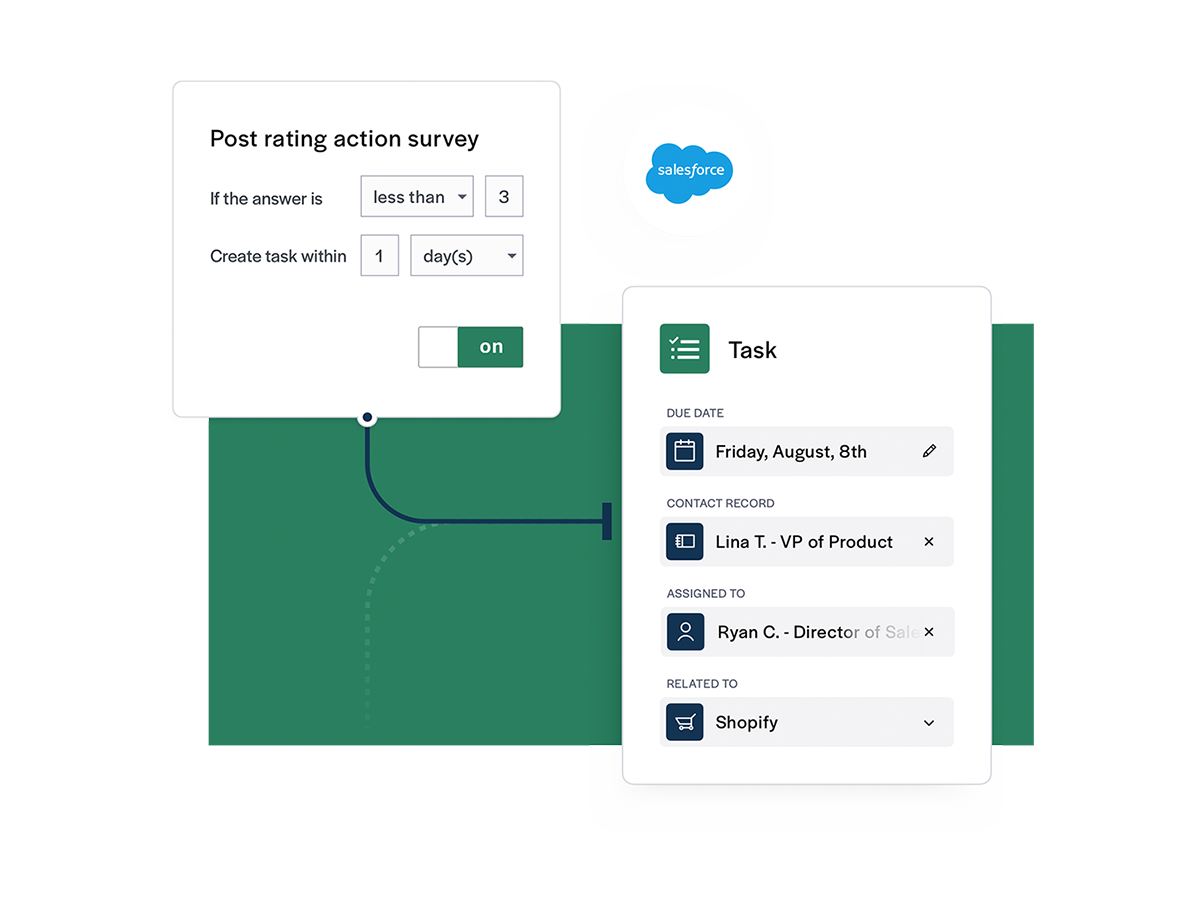In this Salesforce interface screenshot, the background is divided horizontally, with the upper portion in white and the lower portion in green. A blue line diagonally connects two sections: the upper left and bottom right corners of the image. In the top right section of the white background, there is a blue cloud icon with the word "Salesforce" written in white.

In the upper left corner, a white box labeled "Post Rating Action Survey" is displayed. Below this label, the text reads: "If the answer is less than 3." Further below, it specifies: "Create task within one day." These sections contain drop-down boxes, allowing users to modify and input different values.

At the bottom right corner of the image, the interface indicates that the feature is turned on. Directly below, in the green background, a detailed "Task" section is shown. It lists a task with a due date of Friday, August 8th, which is associated with an active record for Lena T., VP of Product, and is assigned to Ryan C., Director. The task is also marked as related to Shopify. Each of these fields is editable, allowing users to update the information as needed.